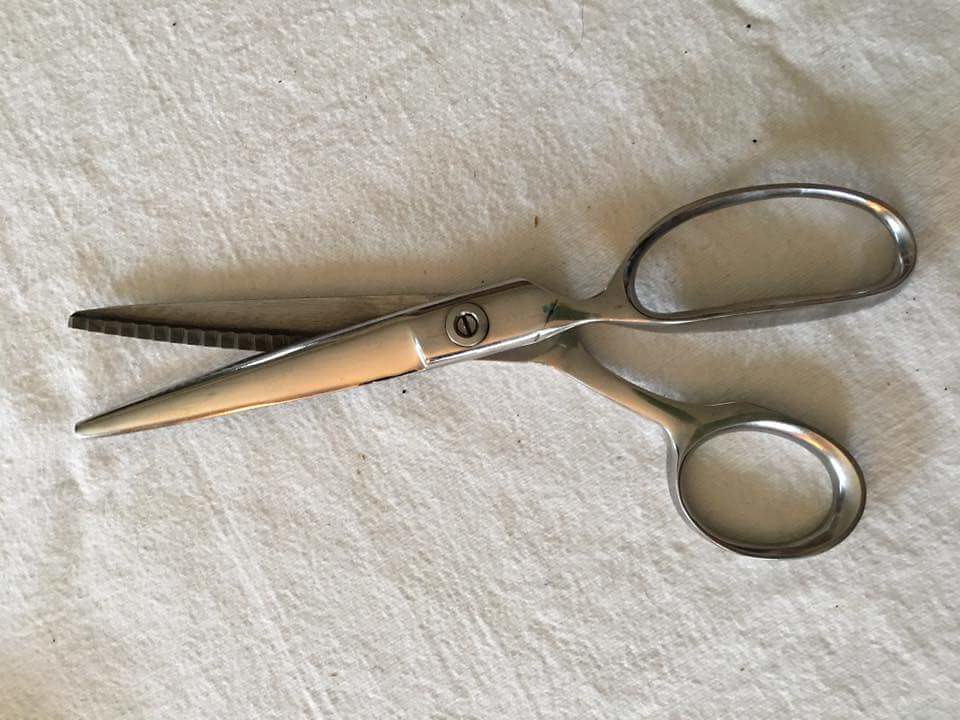Displayed on a piece of textured, white fabric, reminiscent of a flower sack towel, is a pair of silvertone scissors or pinking shears, notable for their slightly worn appearance. The fabric lies beneath the scissors, oriented obliquely and exhibiting visible threads and specks of dirt, contributing to the rustic setting. The scissors, likely made of heavy-duty metal and possibly sterling silver, feature jagged or sawtooth blades rather than smooth ones, indicating they might be used for specialized cutting purposes. They shine under an apparent light source, emphasizing their metallic nature. Positioned with their handle loops on the right and the blade ends on the left, the scissors are slightly open, revealing their aged interior and a visible rivet or screw in the center where the blades cross.